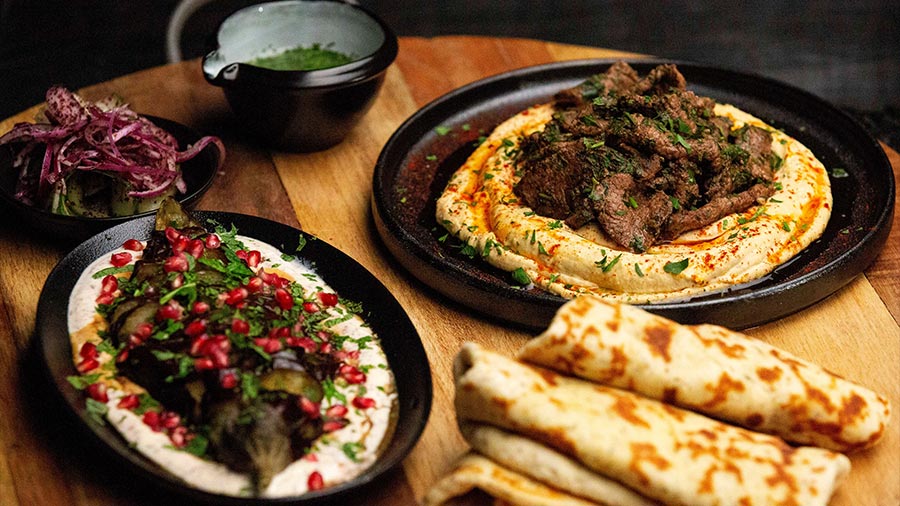This image is a photograph showcasing a vibrant myriad of Middle Eastern dishes arranged on a rustic multi-colored wooden table. At the center, various plates and bowls form a delicious focal spread. To the left, an oval-shaped black plate holds a generous serving of hummus topped with green cilantro and bright red pomegranate seeds. Adjacent to it, another plate displays what looks like a closely garnished dish of hummus crowned with slices of richly cooked beef and sprinkled with fresh cilantro, lying on a bed of orange-tinged hummus drizzled with oil.

In the foreground, a pile of grilled, charred tortillas resembling rolled-up pitas or thick flatbreads are neatly stacked. A black bowl towards the back contains a vibrant green pesto. Next to it, there is a bowl with a pouring lip that seems to contain strips of green onions, hinting at a possible sauce or dressing. Completing the arrangement is a flat dish that appears to be filled with a mix of vegetables such as shredded cabbage or red onion, possibly accompanied by cucumbers or tomatoes. The harmonious composition of robust flavors and textures, highlighted by garnishes like cilantro and pomegranate, vividly illustrates a gourmet Middle Eastern dining experience.